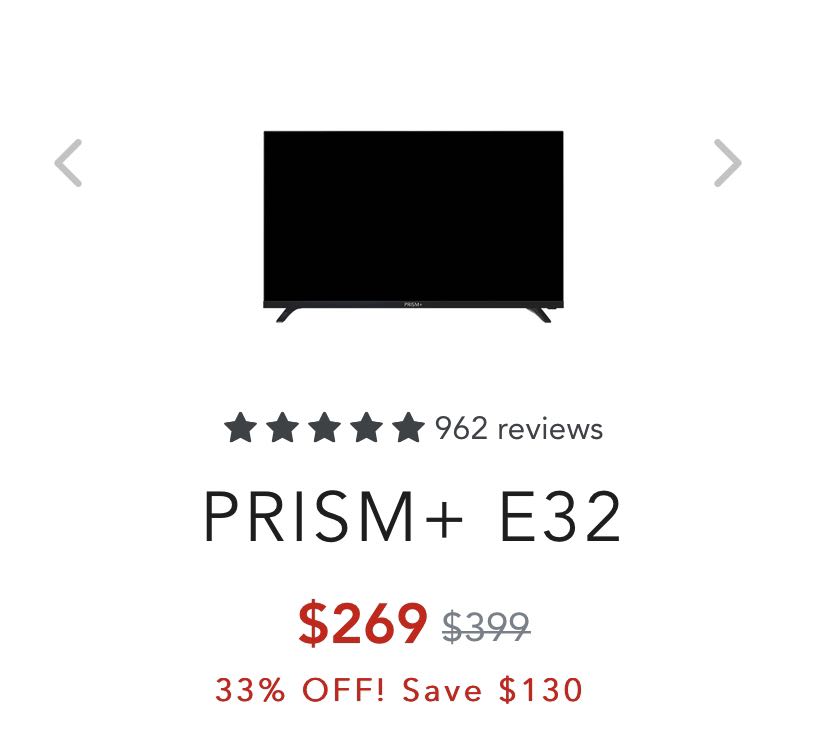The image features a white background showcasing a central banner at the top with left and right navigation arrows. Below the arrows is a prominent black TV set labeled "Prism Plus E32." It is accompanied by five black stars and 962 reviews, indicating a high rating. The TV is priced at $269 in bold red text, marked down from $399, which is shown in light purple with a strikethrough. Additionally, in red text, it announces a 33% discount and a $130 savings.